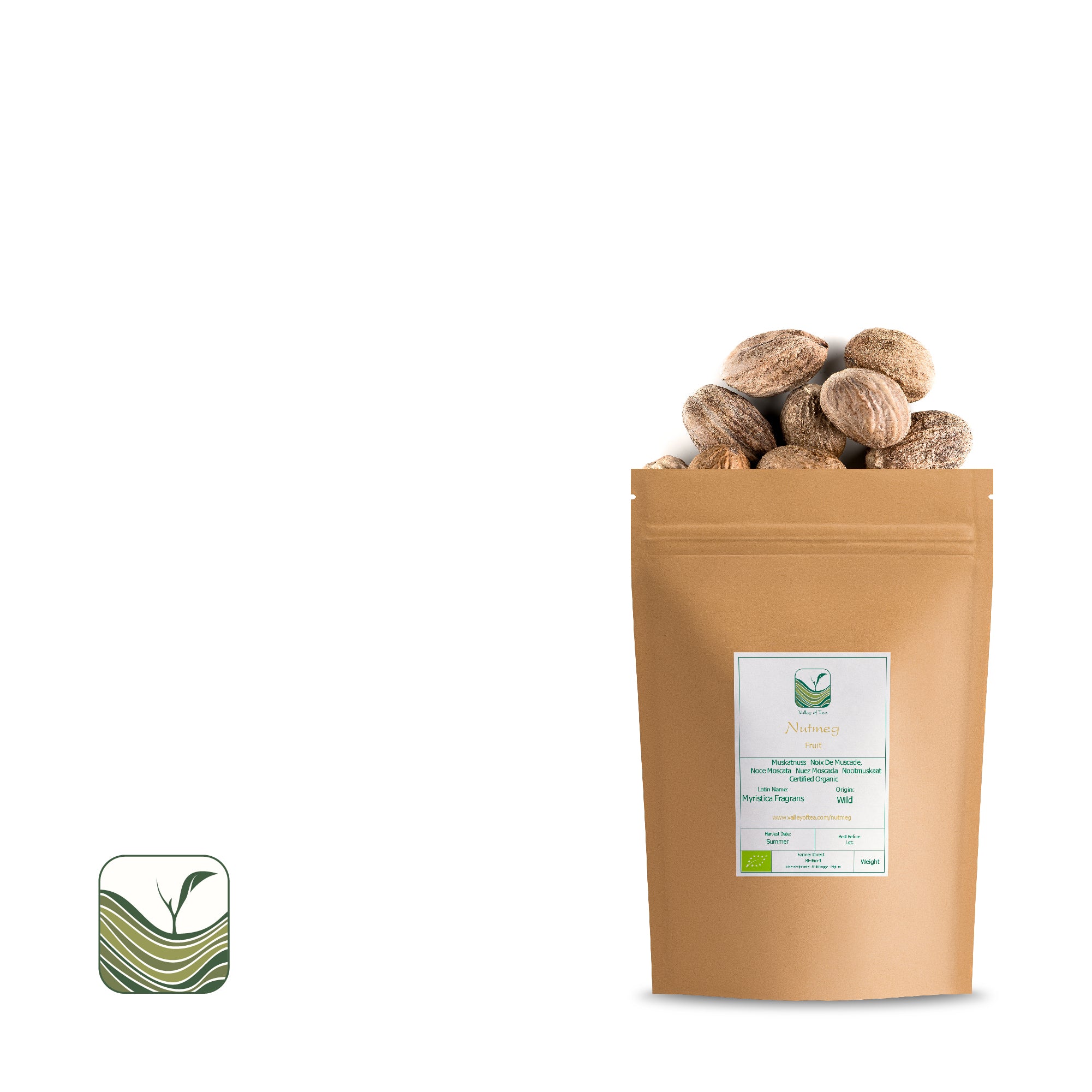This image features a brown, resealable bag of nuts against a white background, with a slight shadow at the bottom. The packaging is light brown, possibly a paper or plastic material, with a small white label in the center displaying green text and an image. The nuts, spilling from the top of the bag, are light brown with darker striations, likely walnuts or nutmeg fruit. On the bottom left corner of the image, separate from the bag, there is a small rounded square logo. This logo includes different shades of green wavy lines at its base and a dark green twig with a single leaf on the right, and another forked twig.